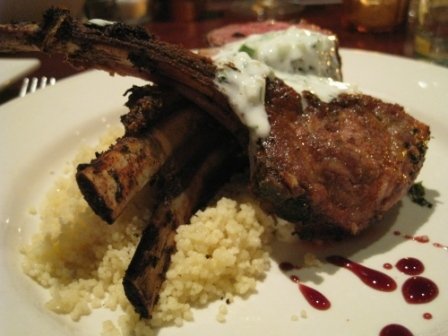In this indoor photograph, a beautifully presented dish is served on a round white china plate, set against a dark, rust-colored table background. The main feature is two well-done lamb shanks crossed artfully, their bones pointing towards the left. The lamb shanks are nestled on a bed of white rice, occupying the left portion of the plate. The meat is adorned with a white cream sauce, likely garnished with chives or scallions, which adds a touch of elegance to the dish. In addition, on the bottom right corner of the plate, a drizzle of reddish barbecue sauce completes the presentation. The surrounding table is slightly visible, hinting at the dining setup with drinking glasses and a fork. The overall scene is a bit dim with a cozy ambiance, and despite the image being slightly out of focus, the meal looks fresh and untouched, ready to be savored.